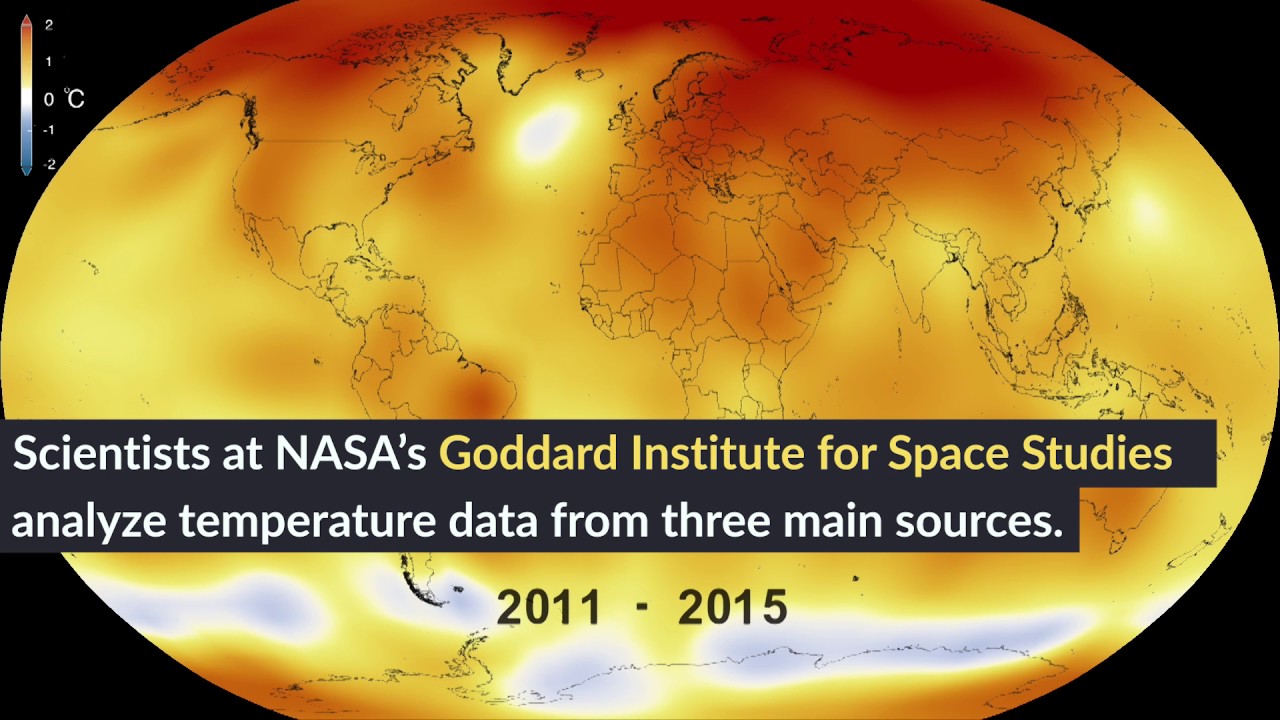This image is a screenshot from a website featuring a predominantly black background. On the upper left side is a multicolored meter. The meter's segments range from dark red at the top to orange, white, light blue, and finally dark blue at the bottom. Adjacent to this meter, numbers are displayed with '2' at the dark red, '1' at the yellow, '0' at the white, '-1' at the light blue, and '-2' at the dark blue. The number '0' is accompanied by a degree Celsius symbol, represented as a large "C".

Prominently in the center of the image is a large oval that visualizes the Earth, depicted in striking colors. The Earth is illustrated in bright orange and yellow hues, with the top exhibiting a dark orange shade. Toward the bottom, various bright white splotches are visible. A notable bright yellow circle with a white center is positioned around the area of Canada.

Overlaying the globe is a banner that reads, "Scientists at NASA, Goddard Institute for Space Studies, analyze temperature data from three main sources." Further, it specifies the time period as "2011 to 2015."